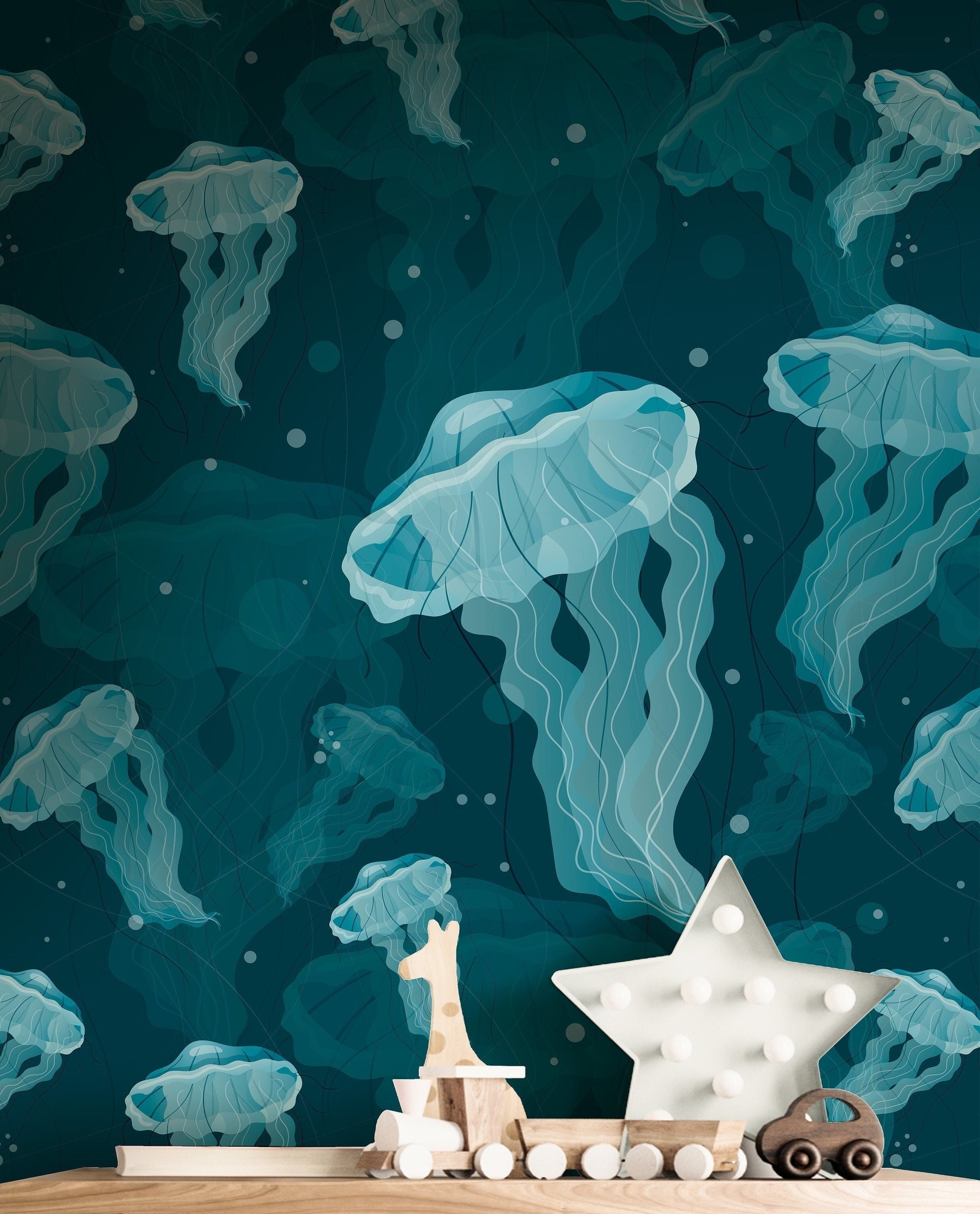This indoor photograph captures a whimsical corner of a child's bedroom. Dominating the background is a dark aqua blue wall adorned with a lively pattern of jellyfish, rendered in lighter aqua and white tones with delicate transparency in some areas, suggesting an underwater scene. Scattered bubbles enhance the marine ambiance. The top portion of a light beige wooden piece of furniture, possibly a nightstand or shelf, is visible at the bottom of the image. Arranged on this surface are various wooden toys: a train with two carts, each sporting white wheels, a small car, and a tan giraffe with darker brown spots. Adding a touch of warmth and comfort, a white star-shaped nightlight with tiny white bulbs stands among the toys, casting a gentle glow.